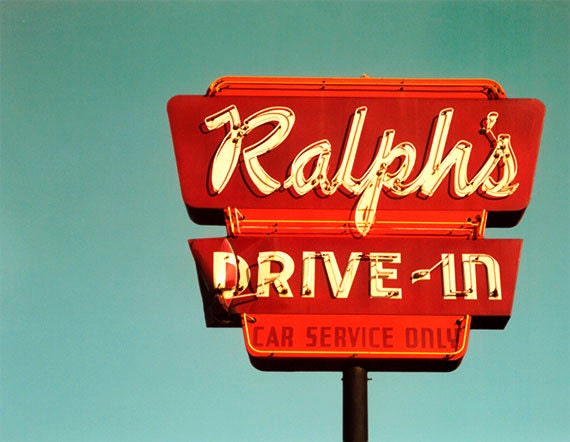The photograph showcases a vintage-style neon sign that evokes a nostalgic 1950s vibe. The sign, primarily red, stands out vividly against a clear medium blue sky, occupying 50% to 75% of the image but positioned off-center. The sign itself is trapezoid-shaped and features three distinct red sections. At the top, in elegant white cursive script outlined in neon tubing, is the word "Ralphs." Below it, in bold, white print also outlined in neon, it reads "Drive-In." Further down, another section of the red sign displays "Car Service Only" in plain red lettering. The sign is mounted on an aged black metal pole and appears worn, with noticeable damage such as a curled and rusted corner near the letter "D" in "Drive-In." The photo, likely taken by a professional from the ground looking up, has enhanced contrast to emphasize the vibrant colors and clear details of both the sign and the sky.